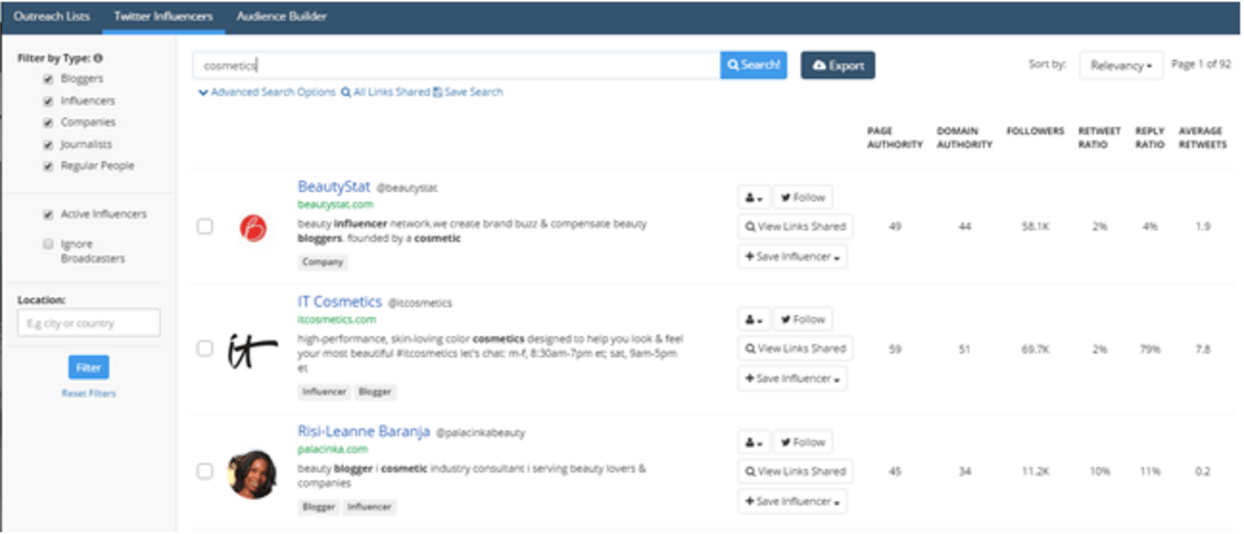The image depicts a social media monitoring and enhancement application interface. Despite its low resolution and blurry presentation, the layout and elements can be identified with difficulty. The interface features a blue header and a thin blue line running vertically along the top left edge. The header includes the options 'Outreach Users,' 'Twitter Influencers,' and 'Audience Builder,' with 'Twitter Influencers' currently selected, indicated by a blue underline.

The main area displays a filtering section labeled 'Filter by Type,' listing categories such as Bloggers, Influencers, Companies, Journalists, and Regular People, all of which are checked. Below this, an option for 'Active Influencers' is also checked, whereas 'Ignore Broadcasters' remains unchecked. There is a search field under 'Locations' and a 'Filter' button nearby.

On the right side, search results are shown, including entries like Beautystat, IT Cosmetics, and Resilien Baranja, each accompanied by small icons and details that are not legible. Next to these details are checkboxes that are currently unchecked. Further to the right, near the top, are two buttons labeled 'Search' and 'Export.'

Additional options are shown in columns, including 'Sort by Relevance,' with navigation controls indicating 'page one of 92.' The menu headers include 'Page Authority,' 'Domain Authority,' 'Followers,' 'Retweet Ratio,' 'Reply Ratio,' and 'Average Retweets.' For the listed entities (Beautystat, IT Cosmetics, Resilien Baranja), various stats are indicated but are too small to discern clearly. Despite the blur, the layout appears organized and user-friendly.